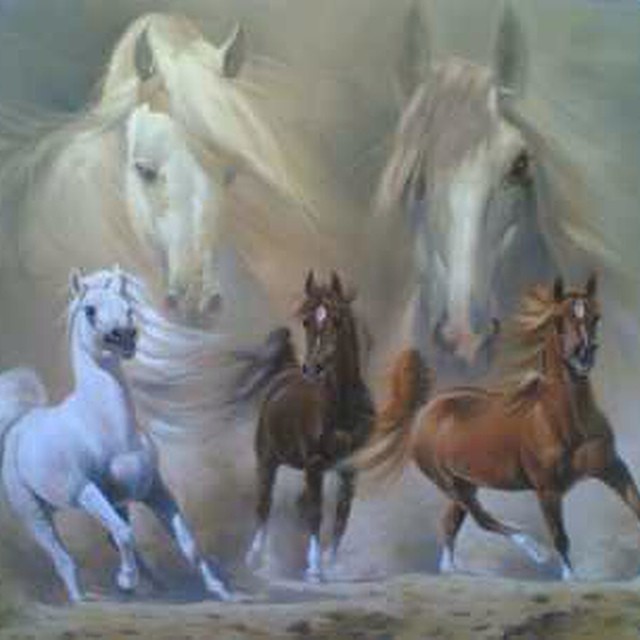This artwork showcases five stylized horses, arranged dynamically across the canvas, evoking a sense of movement and grace. The top half of the piece features the prominent heads of two larger horses, their serene eyes and flowing manes captivating attention. The horse on the upper left is a majestic white with a matching mane, while the one on the upper right sports a pale gray coat and a slightly darker mane with a touch of blonde.

In the foreground, three smaller yet intricately detailed horses are depicted in mid-gallop. A striking pure white horse leads the charge, its mane and tail billowing behind it. Flanking it are two brown horses; the darker one is a chocolate brown with distinctive white "socks" on its legs and a white star on its forehead, while the lighter reddish-brown horse also features white boots and a similar white star, complemented by a flowing mane.

These horses appear to run on a ground surface, seemingly tailed by the ethereal presence of the larger horses above, perhaps symbolizing ghostly ancestors or guardian spirits. The overall composition, likely crafted in watercolors or pastels, emphasizes soft, delicate colors and lines, creating an enchanting, semi-realistic portrayal often seen in horse-themed artwork and decor.